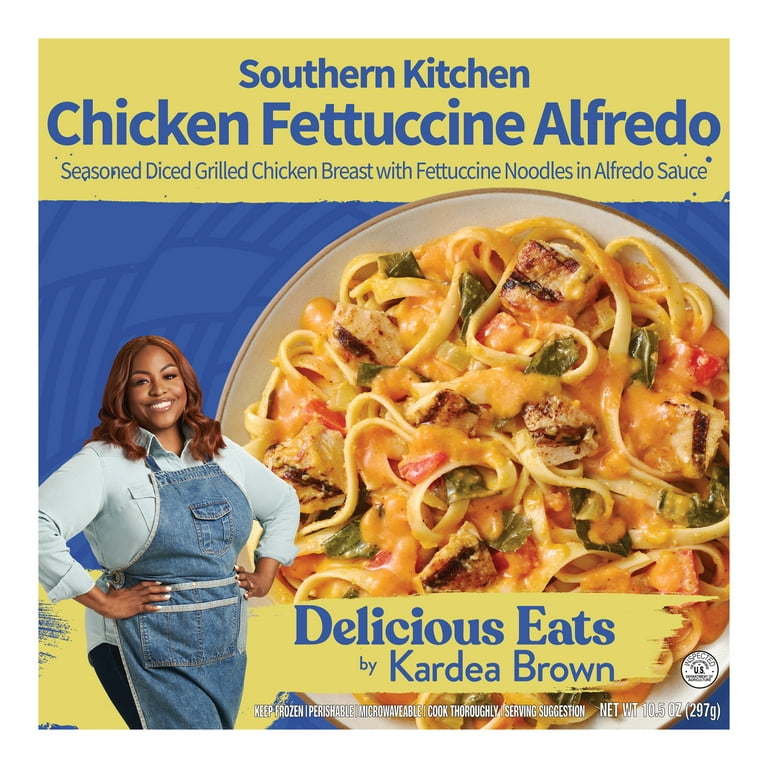The image showcases the packaging for a microwavable meal titled "Southern Kitchen Chicken Fettuccine Alfredo," featuring Seasoned Diced Grilled Chicken Breast with Fettuccine Noodles in Alfredo Sauce. Dominating the bottom left-hand corner is a younger black woman, presumably the creator, Carta (or Kendra/Cordelia) Brown, who is joyfully smiling with her hands on her hips. She’s clad in a light blue shirt under a jean-style apron. Her waist-length reddish-brown hair complements her friendly demeanor. The packaging background is predominantly blue, with yellow-striped borders at the top and bottom containing blue text with the product name and description. A vivid image of the meal itself, showing well-cooked chicken, appealing fettuccine noodles, and colorful peppers, is prominently displayed. Additional text underscores the product’s quick and convenient preparation, indicating it should be kept frozen, is perishable, and should be microwaved thoroughly, with a net weight of 10.5 ounces or 297 grams.